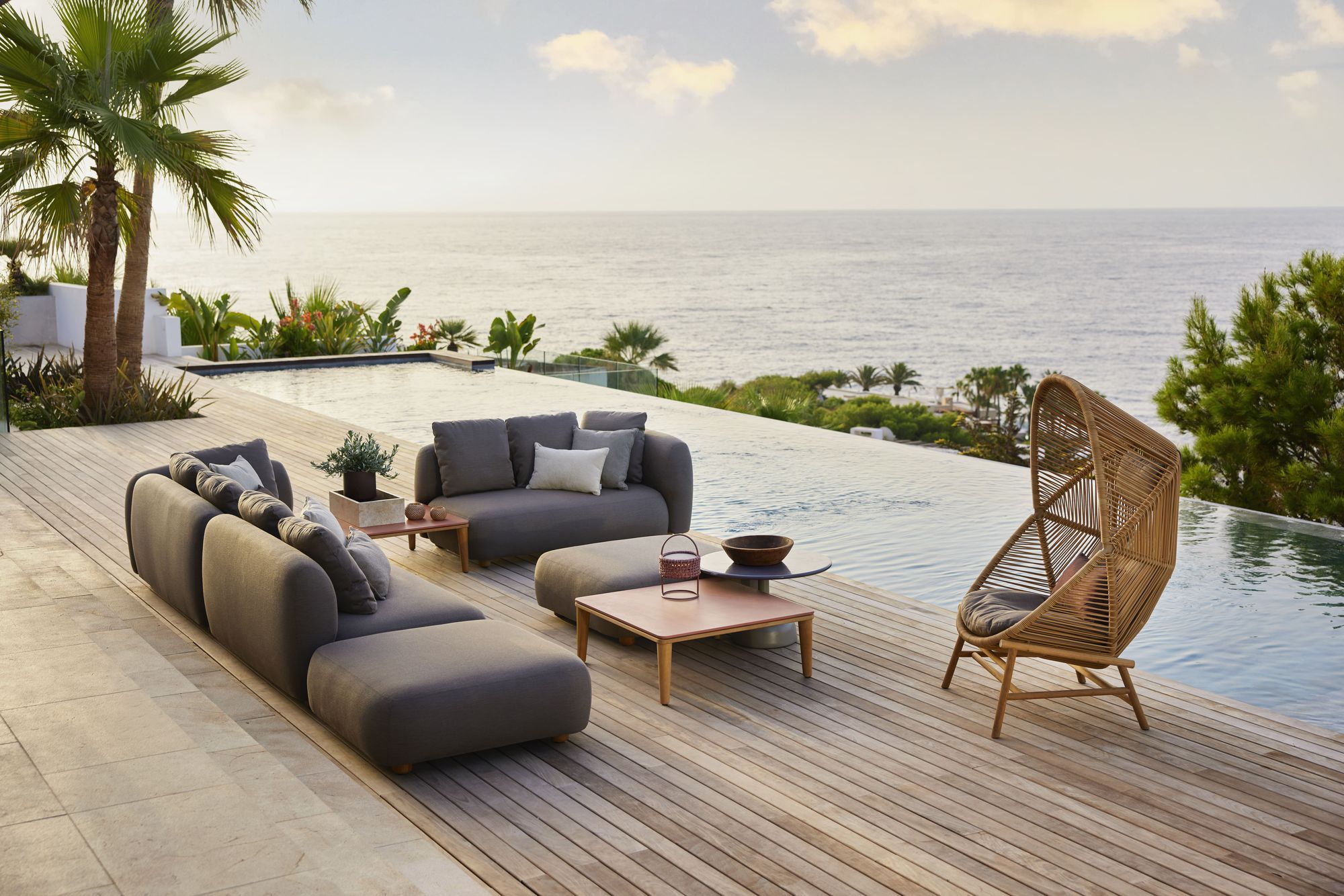This photographic image captures a luxurious outdoor setting on a sprawling hardwood patio that overlooks the vast, serene ocean under a bright blue sky scattered with fluffy white clouds. The focal point is a long, unoccupied infinity pool that stretches along the right side of the deck, seamlessly blending into the horizon. Elegantly arranged around the wooden deck are multiple pieces of sophisticated outdoor furniture. 

On the left side of the image, a gray outdoor sofa with three cushions and several throw pillows faces slightly to the right and away from the viewer. Adjacent to it is a similarly styled loveseat with matching cushions and pillows, oriented towards the first sofa. Between these seating arrangements is a small table adorned with a green plant and two decorative bowls. In front of the loveseat sits a gray ottoman and a compact wooden coffee table bearing a bowl. 

Off to the right side of this cozy seating area stands a wicker easy chair with a cushion and a shaded canopy cover, perfect for relaxed lounging. Another short, round table with an additional dish is positioned nearby. The patio also features a palm tree, planted directly into the decking, and a patch of lush green grass that adds a touch of nature to the polished design. 

In the background, behind the luxurious pool and stylish furnishings, a breathtaking view of the ocean stretches out to meet the sky, with the tops of trees visible just above the wicker chair, completing this idyllic outdoor retreat.